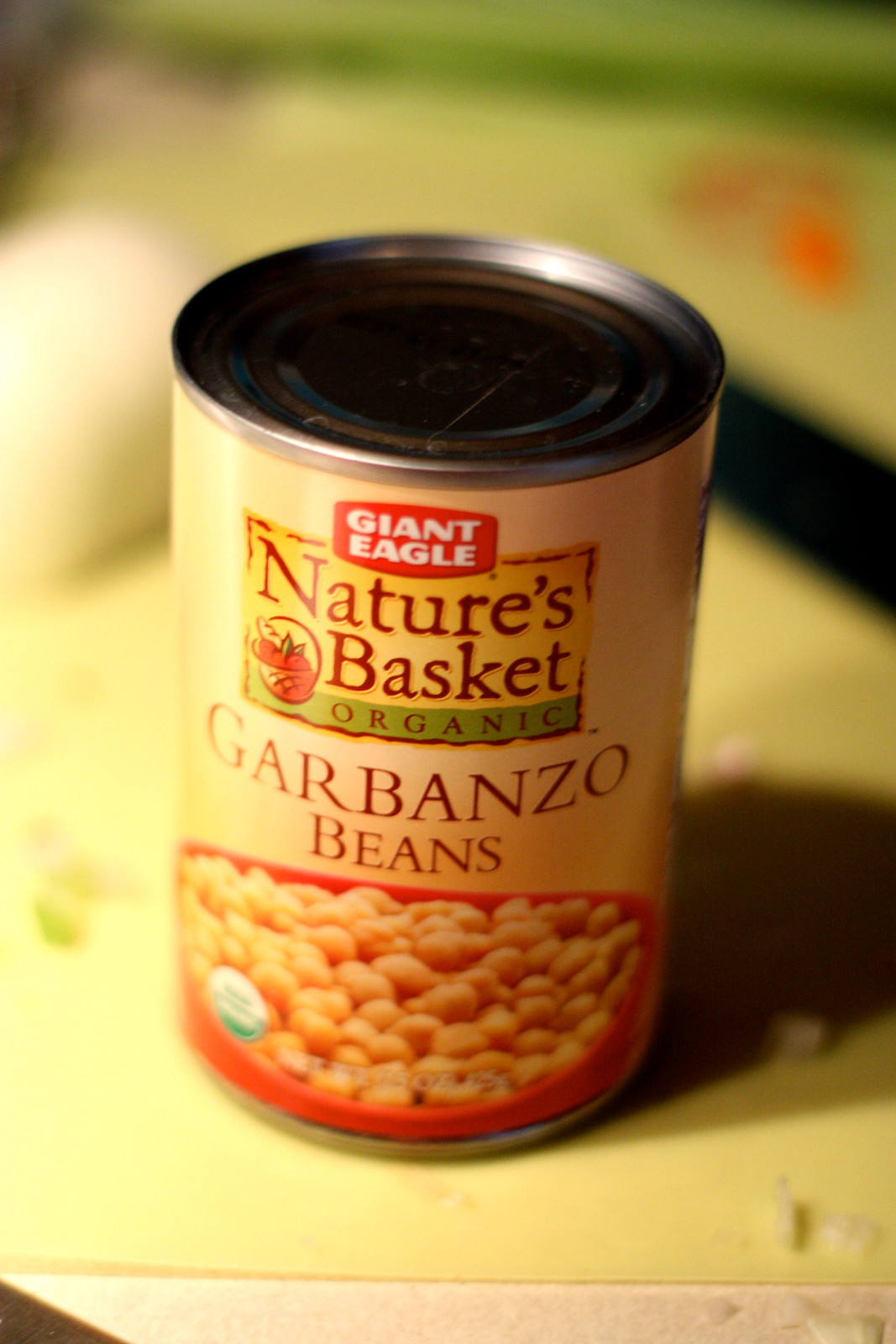This image showcases a close-up of a can of garbanzo beans, prominently displaying its detailed label. At the top, in white text on a red block, it reads "GIANT EAGLE." Below this, the "NATURE'S BASKET" logo is set against a dark yellow background with black text, accompanied by a small basket icon to the left. A green band underneath features the word "ORGANIC" in black lettering. The label then specifies "GARBANZO BEANS" in bold black letters. Below this description, the label depicts the beans, which are orange and set in a red bowl. The can itself has a light brownish hue with the silver aluminum top peeking out. The can rests on a kitchen counter, possibly a cutting board, with what seems to be partially blurred remnants of chopped onion and some indistinct green and orange items visible in the background.